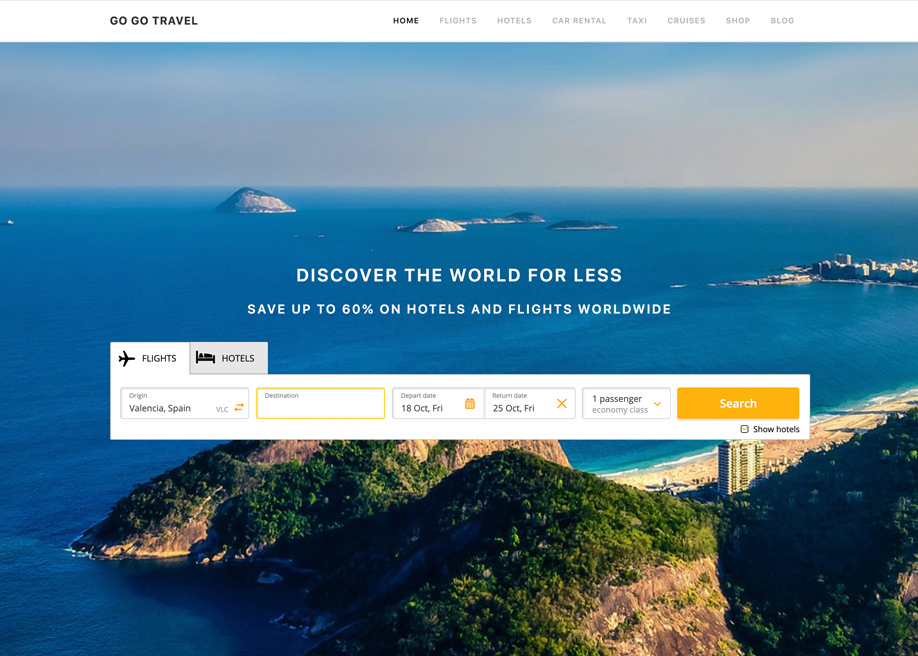A website screenshot for GoGoTravel features a clean, white background with a stylish black header that includes navigation submenus: Home (in black), Flights, Hotels, Car Rental, Taxi, Cruises, Shop, and Blog (all in gray). Dominated by a large, enticing ocean view image, the central portion of the site grabs attention immediately. The serene scene includes a dazzling blue ocean dotted with tan islands crowned with lush greenery. The light ripples on the water surface and the adjoining high-rise buildings flanked by smaller structures create a harmonious blend of nature and civilization.

At the heart of this inviting image, a bold white text says, "Discover the World for Less," promising savings of up to 60% on hotels and flights worldwide. Beneath this promise, a white and gold interactive search box with black font offers options for Flights and Hotels, displayed alongside corresponding icons—a flying airplane and a bed with a person in it. The search form details an itinerary starting from Valencia, Spain, with unspecified destination highlighted in orange, departure set for Friday, 18th October, and return for Friday, 25th October, meant for one passenger traveling in economy class. An eye-catching orange and white search button labeled "Show Hotels" invites immediate action.

The picturesque backdrop, featuring a gorgeous ocean view under a blue sky, interspersed with idyllic islands and bordered by sandy beaches, adds a layer of wanderlust and adventure to the practical search tools of the travel website.